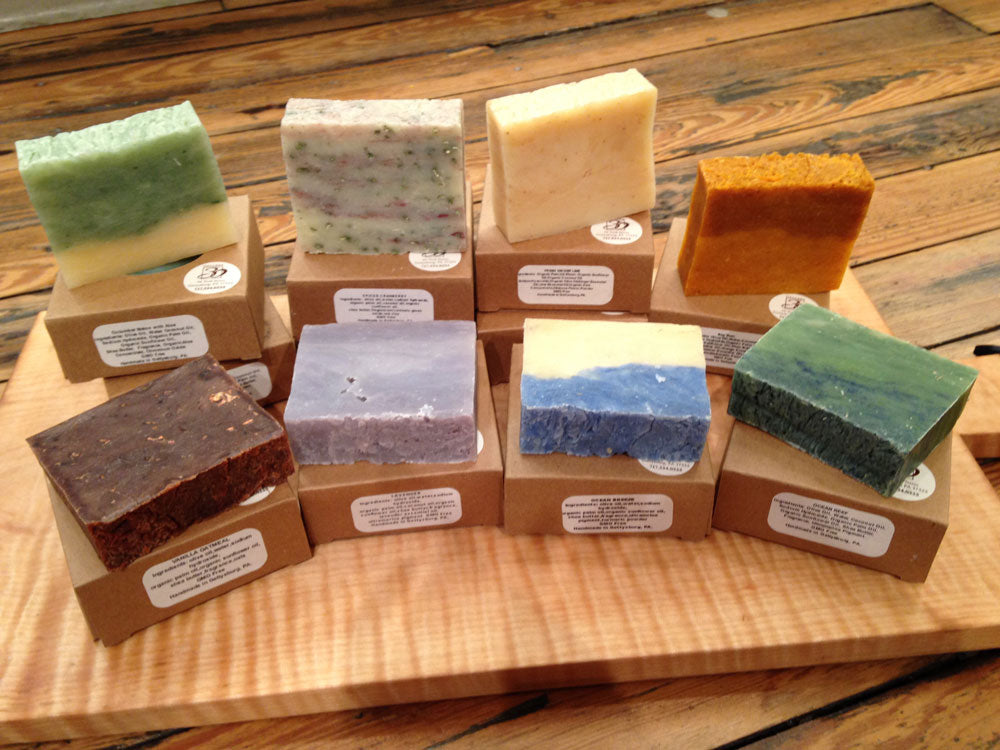The image displays a carefully arranged collection of colorful bars of soap, set on a wooden panel on a wooden floor. The soaps are organized into two rows of four bars each. All the soaps have been taken out of their respective cardboard boxes. Each box is brown with a white rectangular label featuring black text, possibly illustrating the brand's logo and product details. 

In the back row, from left to right, the first soap is a vibrant lime green with whitish tones, followed by a cream-colored bar with red and green specks. Next is a tan-colored soap, and finally, a soap bar with dark orange on top and light orange on the bottom. 

In the front row, starting from the left, there is a chocolate-colored bar, an aqua-blue soap, a two-tone bar with yellow on the top and blue on the bottom, and a dark green soap. These bars of soap are displayed upright, providing a clear view of their surfaces and vibrant colors.